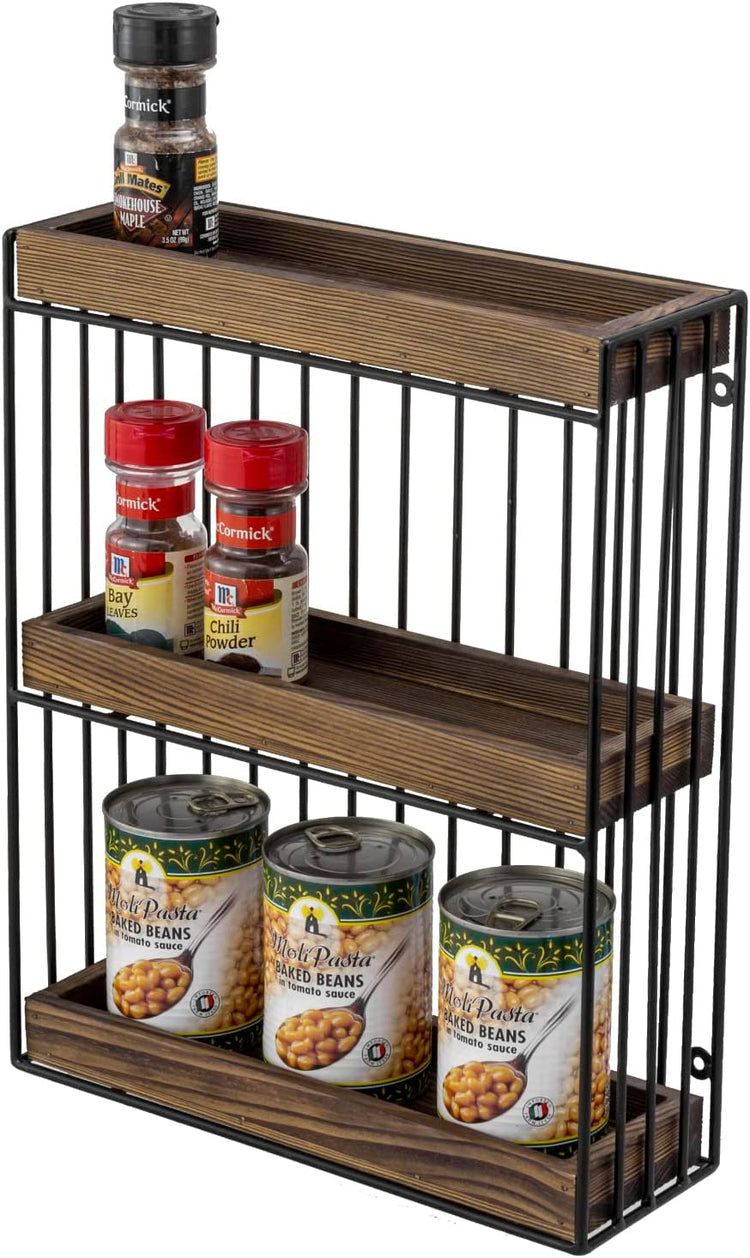This is a detailed product image of a three-tiered spice rack, set against a completely white background to maintain focus on the object. The rack features three shelves constructed from medium dark brown wood, securely held together by robust iron metal vertical bars on the sides that extend from the top to the bottom, as well as bars that frame the top and bottom. 

The bottom shelf is fully occupied by three cans of baked beans in tomato sauce, each bearing a pop-top lid, with labels depicting a spoon filled with beans. The middle shelf holds two McCormick spice jars: one containing bay leaves and the other chili powder, both distinguished by their red caps. The top shelf features another McCormick spice jar, specifically the Smokehouse Maple variety of steak seasoning. Additionally, the back panel is made of black wire with holes for wall mounting, reflecting the spice rack's practical design intended for both countertop use and wall attachment.